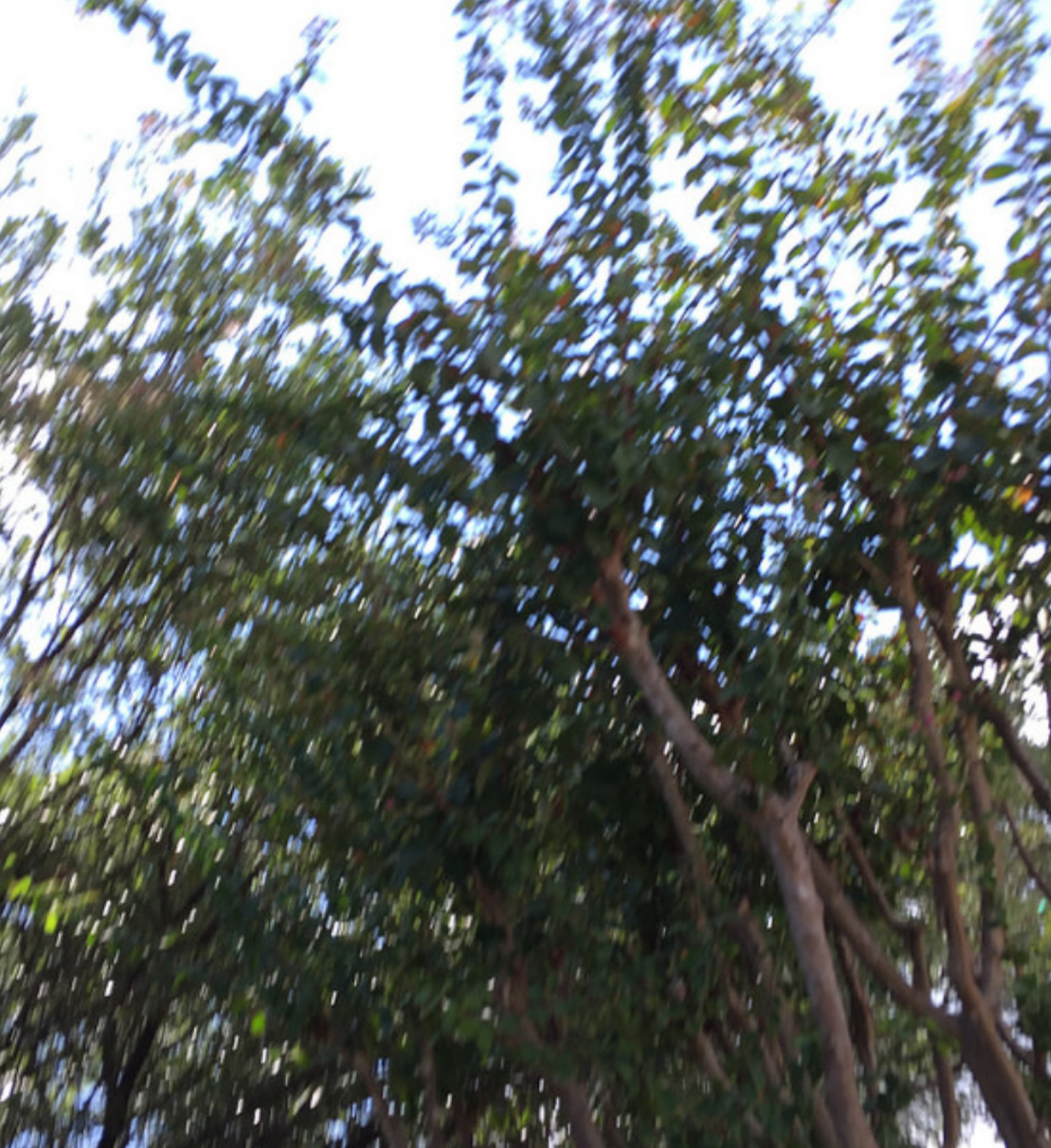The outdoor daytime photograph captures a dramatic upward view of several mature trees dominating the frame. The camera is angled at roughly 45 degrees, emphasizing the reach of the branches that extend high into the brilliantly overexposed sky, which appears as a uniform white due to the lighting. The dense foliage primarily consists of dark green leaves, with some lighter green areas where light filters through. Amidst the verdant canopy, patches of yellowish-brown and occasional red leaves are visible, adding a touch of varied color. The branches, which emerge from the bottom right corner and stretch upwards, are uniformly brown with lighter knots. The image has a slightly blurry quality and lacks distinct focus, giving it a dreamy, almost ethereal atmosphere. Overall, the photograph showcases the intricate interplay of tree trunks, branches, and leaves against a stark white sky.